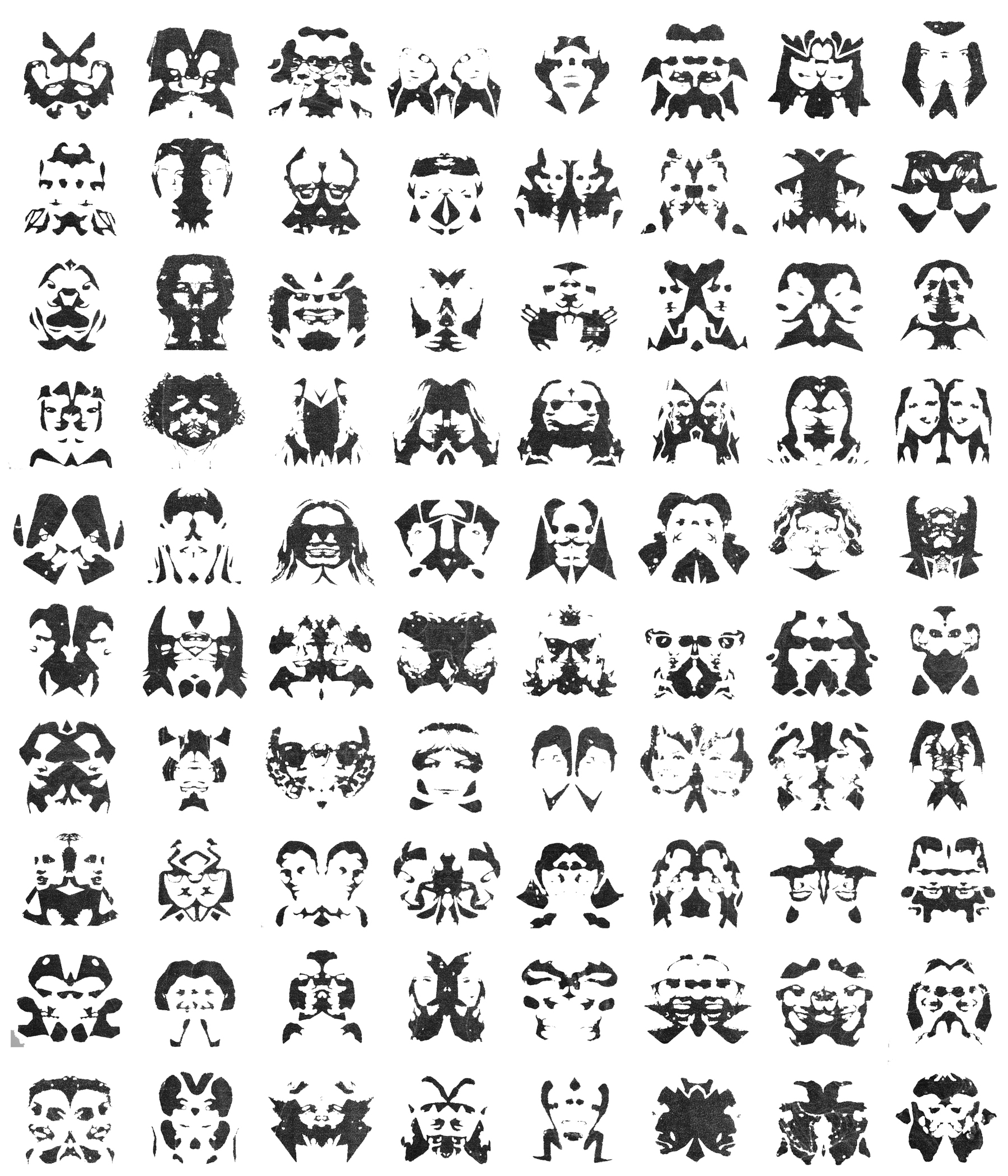This image features a white background with a grid of 80 black-and-white stamped faces arranged in 10 rows across and 8 rows down. Each face is mirrored, creating a doubled or folded appearance that gives a slightly surreal and distorted look. The mirrored effect results in some faces with clearly separated duplicate features, such as two sets of eyes, noses, and mouths, while others have overlapping features that blend together, making it hard to distinguish individual facial elements. The faces are quite detailed despite their small size, though it's challenging to discern if they belong to actual people or if they are abstract representations. The repeated faces add to the complexity and visual interest of this art piece.